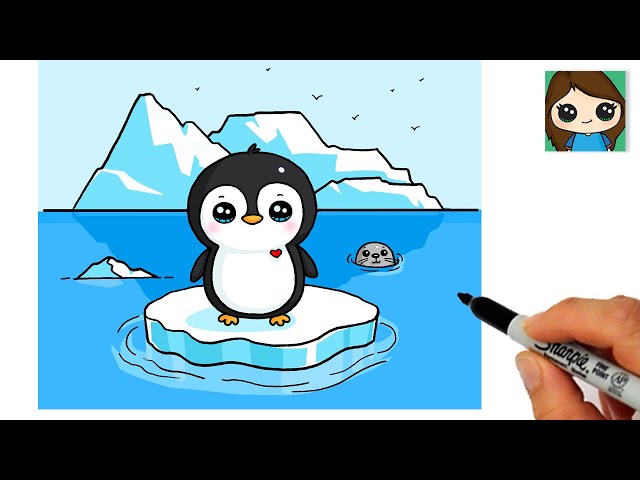The image is a detailed, cartoonish drawing centered on a very cute baby penguin standing on a misshapen piece of floating ice in a serene, light blue ocean. The baby penguin, which is mainly black with a white face and underbelly, features large, watery black eyes and a small red heart on its upper left chest. To the right, just behind the penguin, a light gray seal’s head peeks out of the water. The background showcases a large land mass of icebergs in shades of turquoise blue with white highlights and a clear blue sky above, dotted with a few black birds. Adding a meta touch, in the bottom right corner, there is a white person's hand holding an uncapped, black Sharpie marker, suggesting the drawing was recently completed. In the top right corner, a small cartoon image of a girl is also visible.